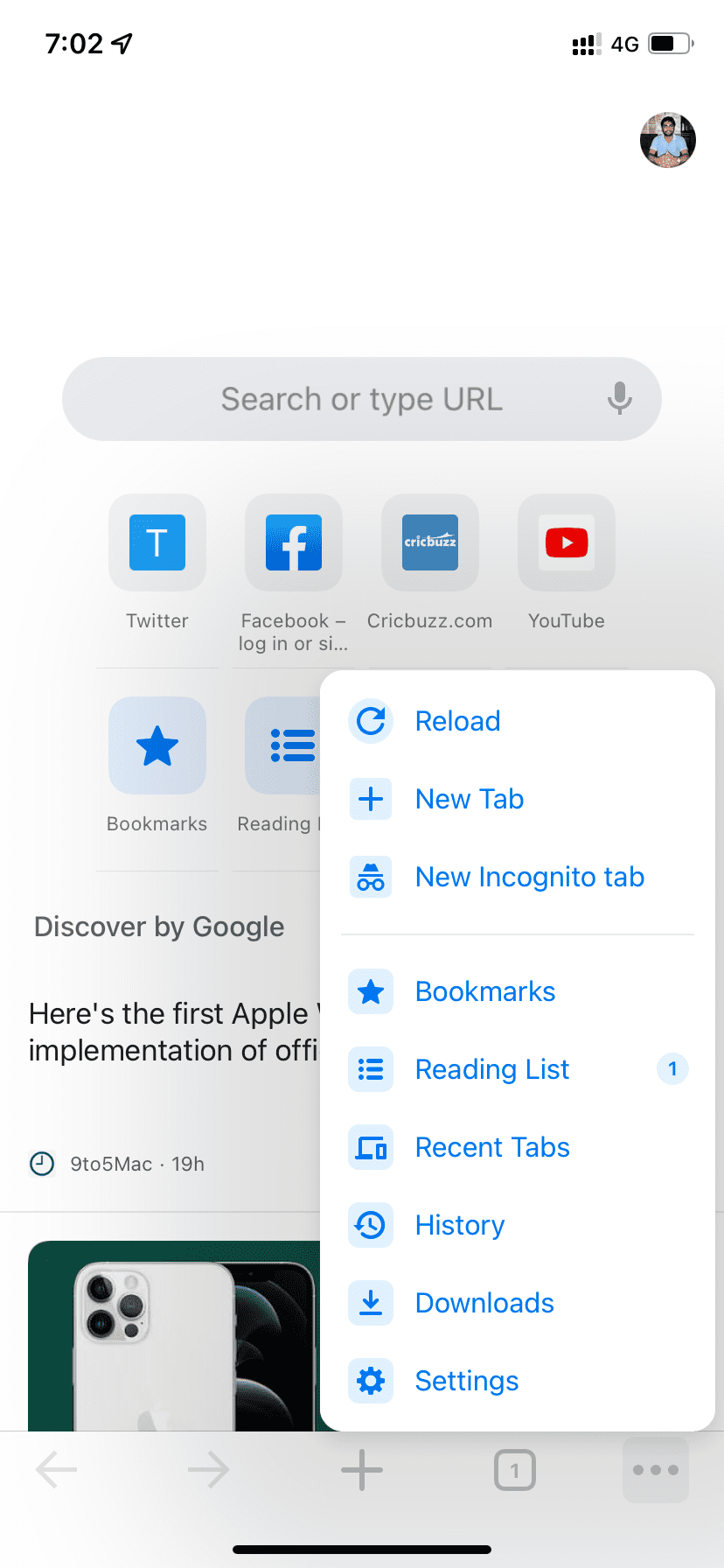The image is a screenshot of a web browsing interface on a mobile device. At the top of the screen, there's a status bar displaying "4G" connection, a partially filled battery icon, and the time "7:02". Below the status bar, there is a gray search bar labeled with "Search or type URL" with a small person icon situated beneath the battery indicator.

Directly underneath the search bar are quick access icons for popular websites: "Twitter" (represented by a 'T' symbol), "Facebook" (with the Facebook logo), "Crickbuzz" (displayed within a blue box with writing), and "YouTube" (signified by a red box with a white triangle). Following these icons, the screen displays the words "Bookmarks" and "Reading List".

A pop-up menu is also visible in the screenshot with a white background. The menu options include "Reload," "New tab," "New incognito tab," and are separated by a line from additional options: "Bookmarks," "Reading list," "Recent tabs," "History," "Downloads," and "Settings". Next to the "Reading list" option, there's a circle with the number "1" indicating an unread item.

At the lower part of the screen, partially obscured by the pop-up, it says "Discover by Google". The snippet of an article teaser reads "Here's the first Apple..." and "...implementation of office ..." although the full text is not visible due to the pop-up. The source shows "9 to 5 Mac" dated 19 hours ago.

Beneath this text, there is a green background featuring an image of an iPhone, displaying both the front and back views of the device. Further down, there's a series of unidentified icons, followed by a black bar spanning the width of the screen at the bottom.